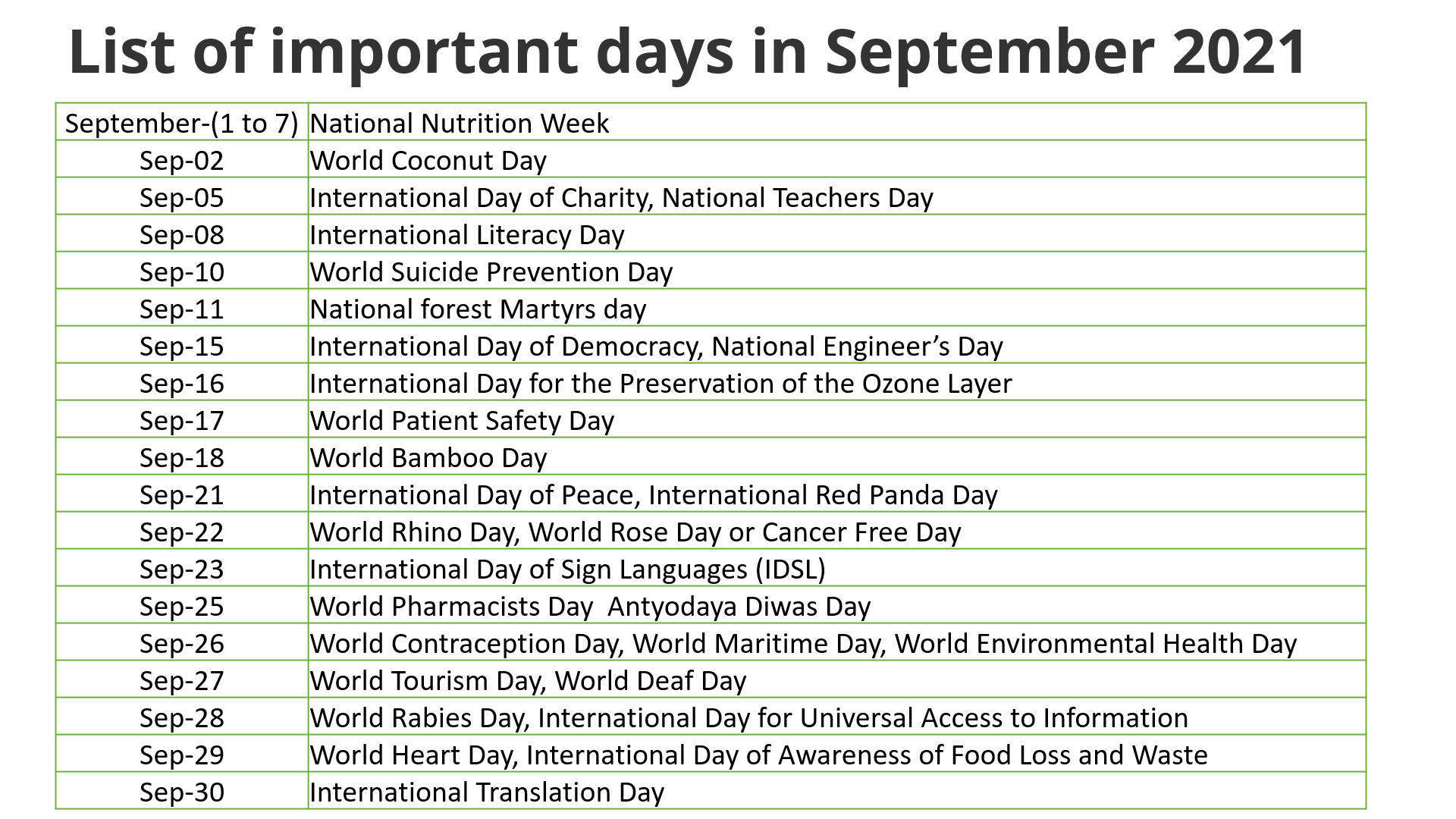The image features a detailed table titled "List of Important Days in September 2021," written in black letters. The table contains a chronological list of significant days celebrated in the month of September, starting from the 1st to the 30th. Each date is associated with specific observances or events, as follows:

- **September 1-7:** National Nutrition Week
- **September 2:** World Coconut Day
- **September 5:** International Day of Charity, National Teacher's Day
- **September 8:** International Literacy Day
- **September 10:** World Suicide Prevention Day
- **September 11:** National Forest Martyrs Day
- **September 15:** International Day of Democracy, National Engineer's Day
- **September 16:** International Day for the Preservation of the Ozone Layer
- **September 17:** World Patient Safety Day
- **September 18:** World Bamboo Day
- **September 21:** International Day of Peace, International Red Panda Day
- **September 22:** World Rhino Day, World Rose Day (Cancer Free Day)
- **September 23:** International Day of Sign Languages (IDSL)
- **September 25:** World Pharmacists Day, Antyodaya Diwas
- **September 26:** World Contraception Day, World Maritime Day, World Environmental Health Day

The table continues to list important observances until September 30th, providing a comprehensive overview of the diverse international and national days observed throughout September 2021.